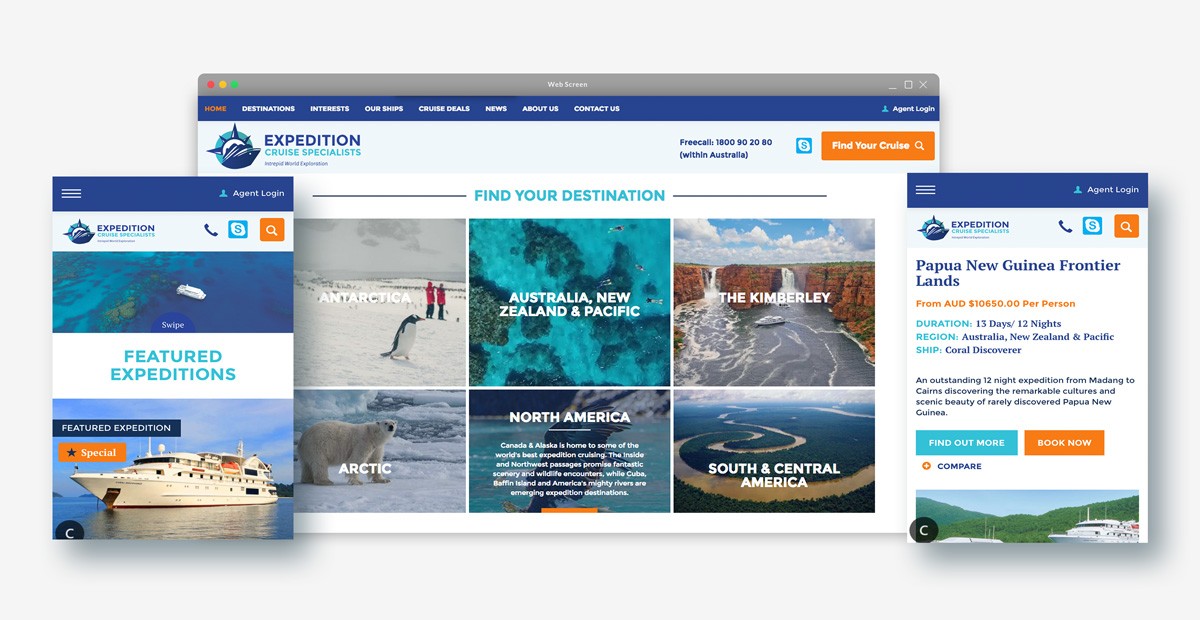The image comprises three screenshots from the same website, identified as "Expedition Cruise Specialist." On the right side of the website, there is a phone number, which appears blurry and is difficult to discern. Prominently displayed on the right is a large, orange rectangular bar with white text that reads "Find Your Cruise."

In the middle section of the page, there is a feature titled "Find Your Destination," listing various expedition destinations including Antarctica, the Arctic, Australia and New Zealand, the Pacific, the Kimberley, South and Central America, and North America.

On the left screenshot, there is a section labeled "Featured Expeditions," showcasing an image presumed to be one of the cruise ships offered by the company. The screenshot on the right highlights a specific expedition titled "Papua New Guinea Frontier Lands," which includes some details about the cruise, though the text is very small and difficult to read.